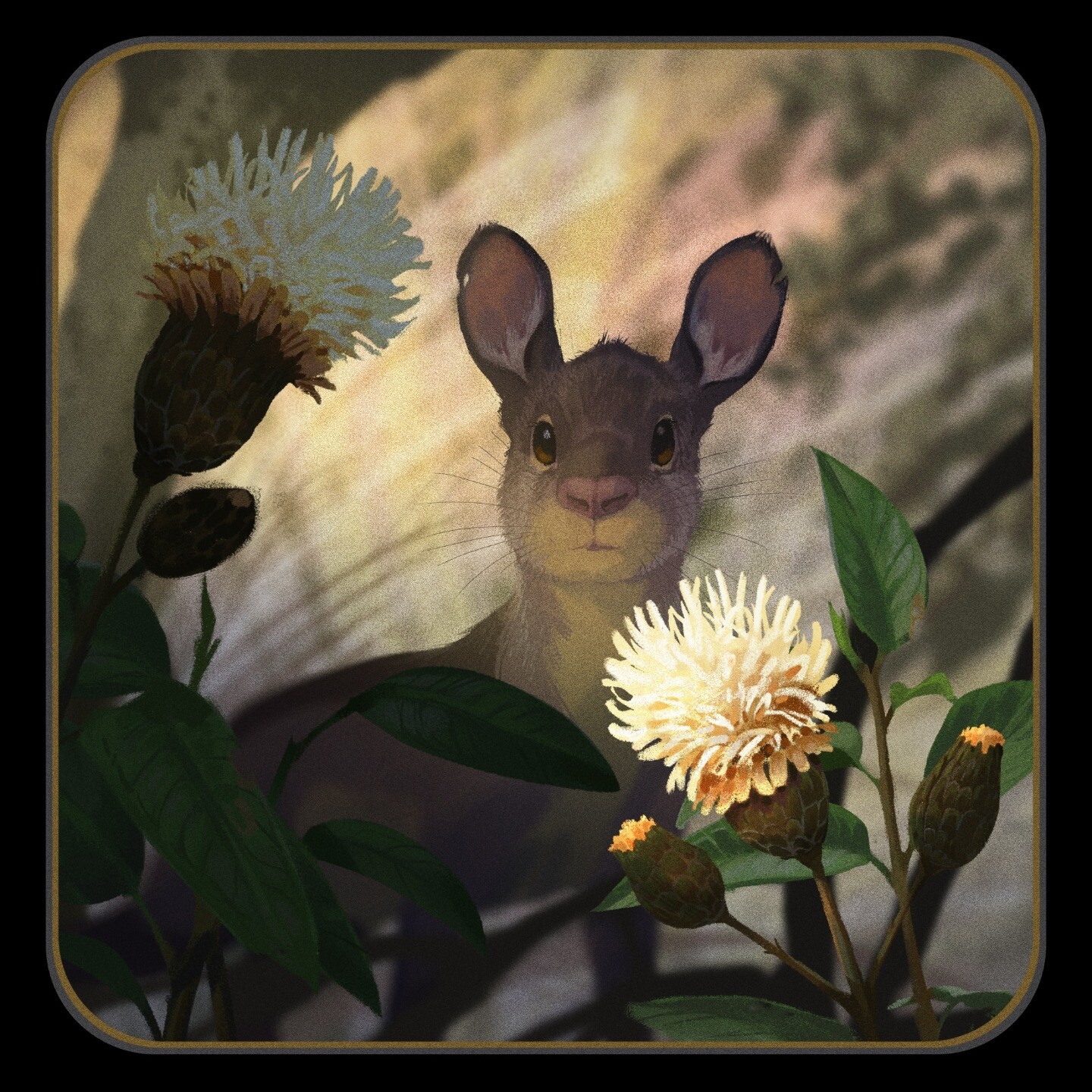In this enchanting AI-generated image, the central focus is a young rabbit, endearingly gazing straight ahead with its large, brown eyes, exuding a sense of curiosity. The rabbit, with its soft gray head, pink nose, and white chest, stands out vibrantly. Its big, oval-shaped ears, which are upright with a pink interior, extend full of life, adding to its overall cuteness. The rabbit's whiskers sprout prominently from its muzzle area, enhancing the intricate details of its face. 

Surrounding the inquisitive creature, a couple of prominent dandelions are showcased. One is fully bloomed with white spores and a subtle yellow base, while two others remain as buds, poised to sprout. These dandelions, along with a lush array of green leaves, create a vivid and colorful foreground against the darker tones nearby. Additional foliage and a muted tree silhouette serve as a soft backdrop, set against a beige-colored background, emphasizing the light and airy feel of the scene. The rabbit's partially obscured back body, hidden behind the leaves, adds a slight air of mystery to the composition. All together, this dynamic and detailed image captures the serene moment of a young rabbit nestled amidst nature's delicate blooms.